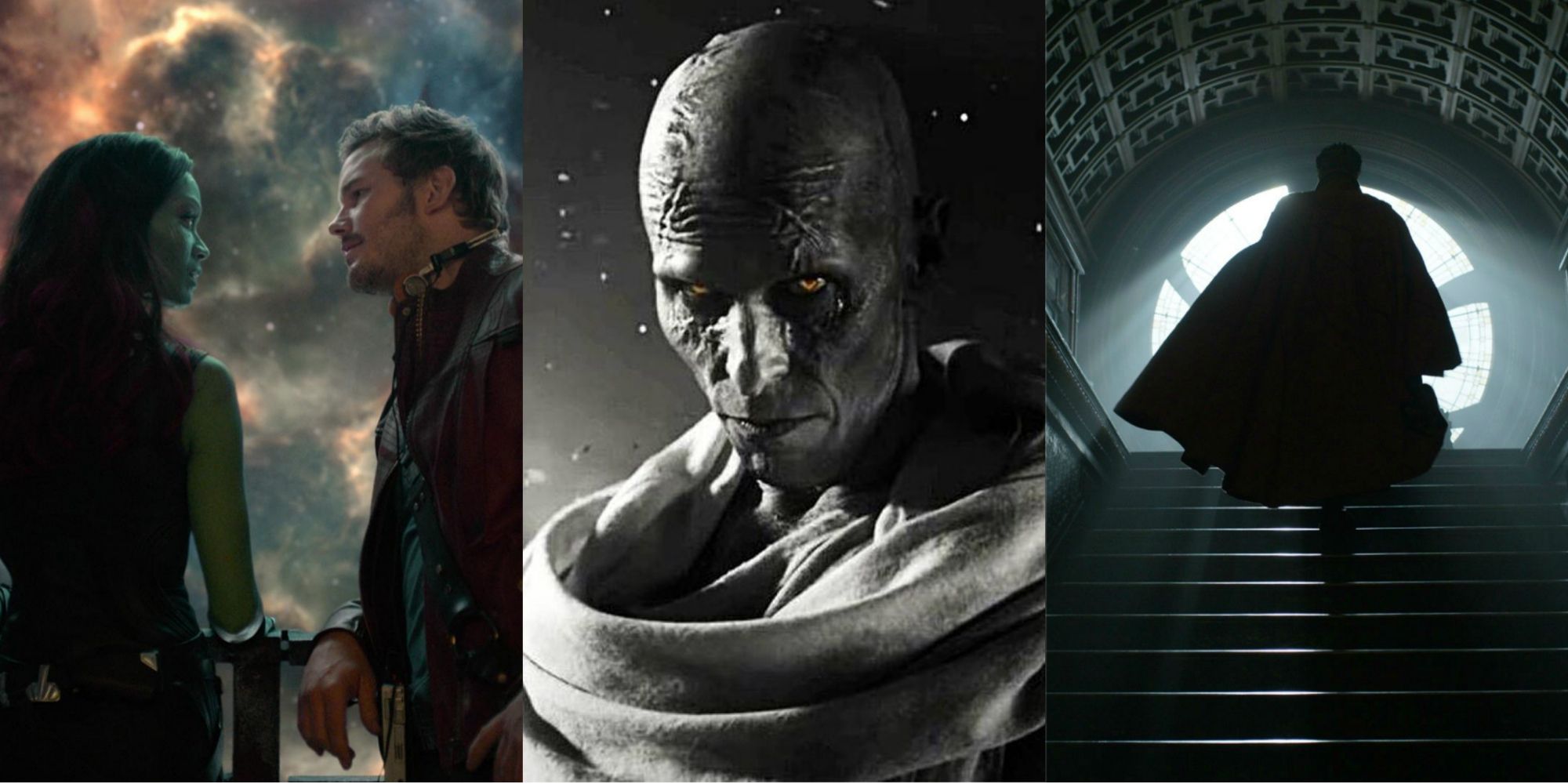This three-part image collage depicts scenes from the Marvel Cinematic Universe, each occupying an equal third of the combined image. The left third captures a moment from "Guardians of the Galaxy," where Gamora, the green-skinned female character, faces Star-Lord (Peter Quill). Star-Lord, characterized by his short brown hair, goatee, and brown leather jacket, stands against a mesmerizing backdrop of a galaxy or nebula, hinting at their cosmic adventures. The middle third showcases a sinister figure from "Thor: Love and Thunder," identified as Gorr the God Butcher, with his distinctive gray skin, ominous runes or scars across his forehead, and striking golden eyes. His presence, accentuated by a large scarf, adds an eerie, otherworldly ambiance. Finally, the right third portrays Doctor Strange, shrouded in his iconic robe, ascending a staircase towards an archway. The scene is set in his headquarters, further emphasized by the dark, mystical atmosphere as he gazes out a window.